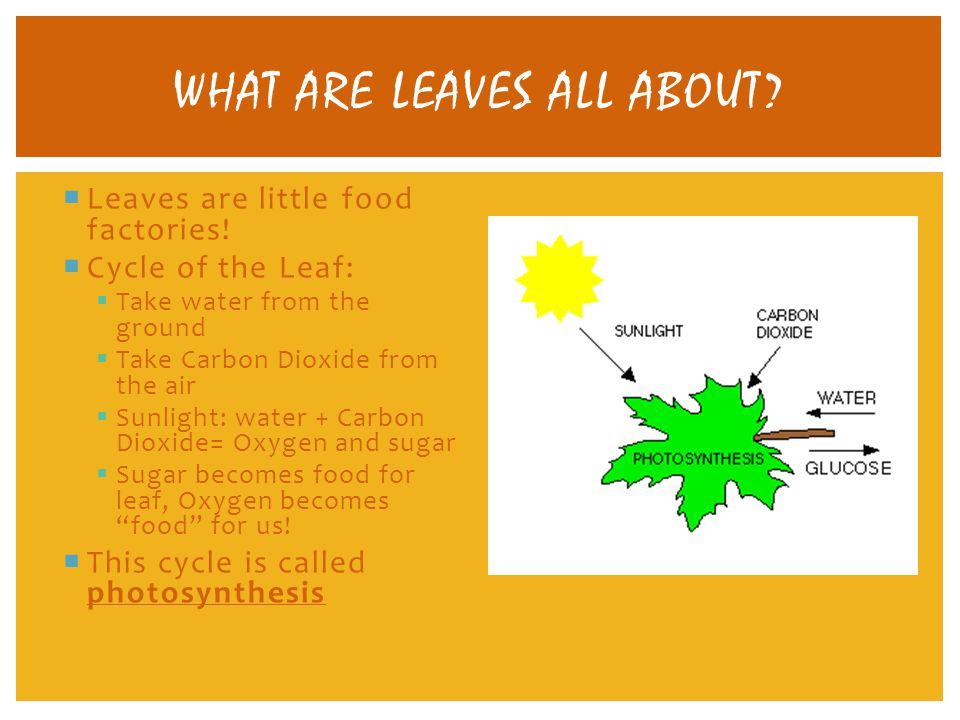The PowerPoint slide features a visually engaging layout designed to explain the process of photosynthesis in a detailed and organized manner. 

The slide has a dark orange title banner at the top, where it prominently displays the title, "What are leaves all about?" Below this, the slide background transitions to a lighter orange.

On the left side, a structured, bulleted list breaks down the information:
- "Leaves are little food factories."
- "Cycle of the leaf," which includes several sub-bullets:
  - "Take water from the ground."
  - "Take carbon dioxide from the air."
  - "Sunlight + water + carbon dioxide = oxygen and sugar."
  - "Sugar becomes food for the leaf."
  - "Oxygen becomes food for us."
- "This cycle is called photosynthesis."

On the right side of the slide, a detailed diagram visually explains the process of photosynthesis. At the center is a depiction of a leaf labeled "photosynthesis." 
- An arrow labeled "sunlight" points from a picture of the sun to the leaf.
- Another arrow labeled "carbon dioxide" directs from the air to the leaf.
- A third arrow labeled "water" points from the ground to the leaf.
- Finally, an arrow marked "glucose" points away from the leaf, indicating the production of sugar.

This combination of textual and visual elements provides a comprehensive overview of the function of leaves and the process of photosynthesis.